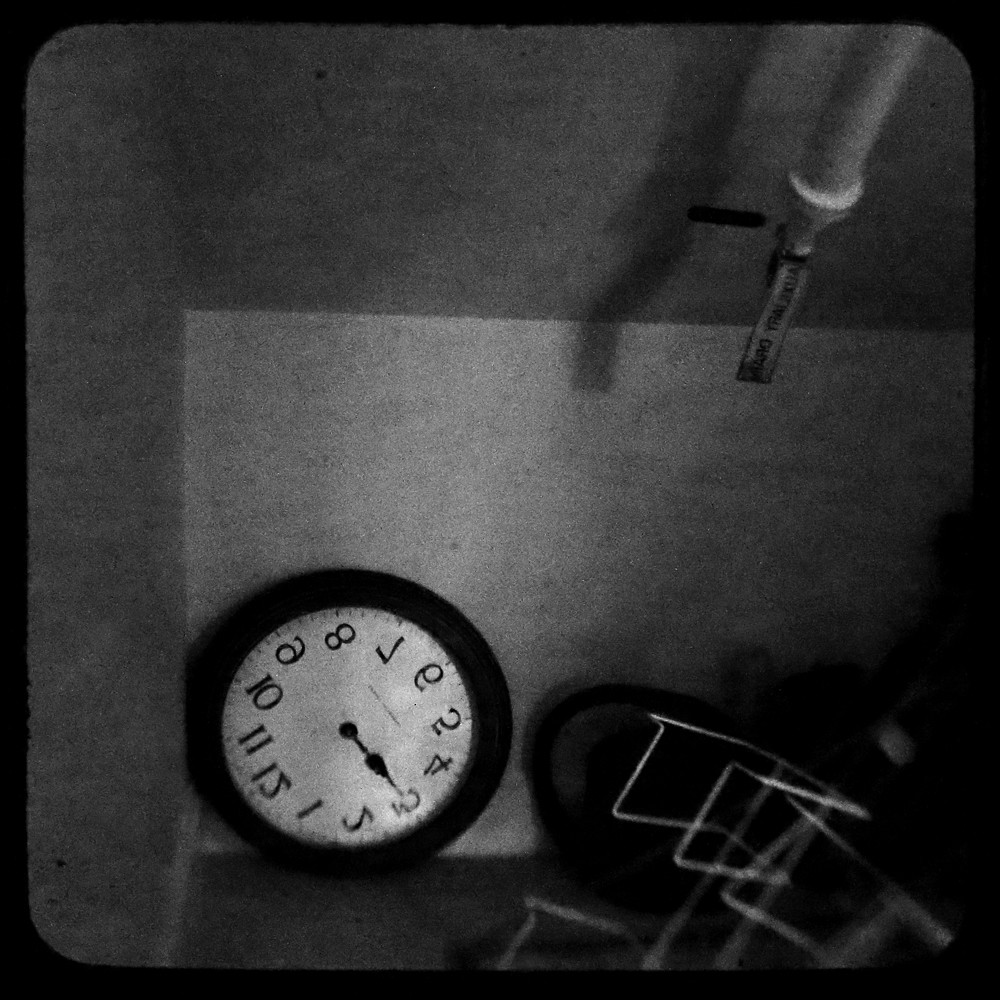This intriguing black-and-white image combines elements of surrealism and abstraction, resembling both a grainy photograph and a meticulously crafted pencil drawing. The entire composition is bordered by a thin, black frame, possibly evoking the edges of a film strip. In the background, a layered geometric pattern is formed with a light gray square encased within a darker gray square, all surrounded by the black frame. The image, which seems to simulate the view inside a box or vessel, contains a variety of objects that blend everyday familiarity with abstract confusion.

At the bottom left corner of the image sits a round clock with a black circular border. Inside its frame, the clock face appears light in color, with numbers that are peculiarly reversed as if seen in a mirror. The hands of the clock point to the two, adding to the enigmatic nature of the scene. To the top right, a pipe-like cylindrical object with a thinner metal extension casts a shadow across the enigmatic space. This pipe appears white against the dark backdrop. 

Additionally, at the bottom right, a blurry, white, squiggly structure is visible, possibly resembling a metal arch or mini dish drainer, though its exact nature remains ambiguous. This object, too, seems to be interacting with reflections within the box-like environment. The entire portrayal compels the viewer to ponder its abstract and mysterious essence.